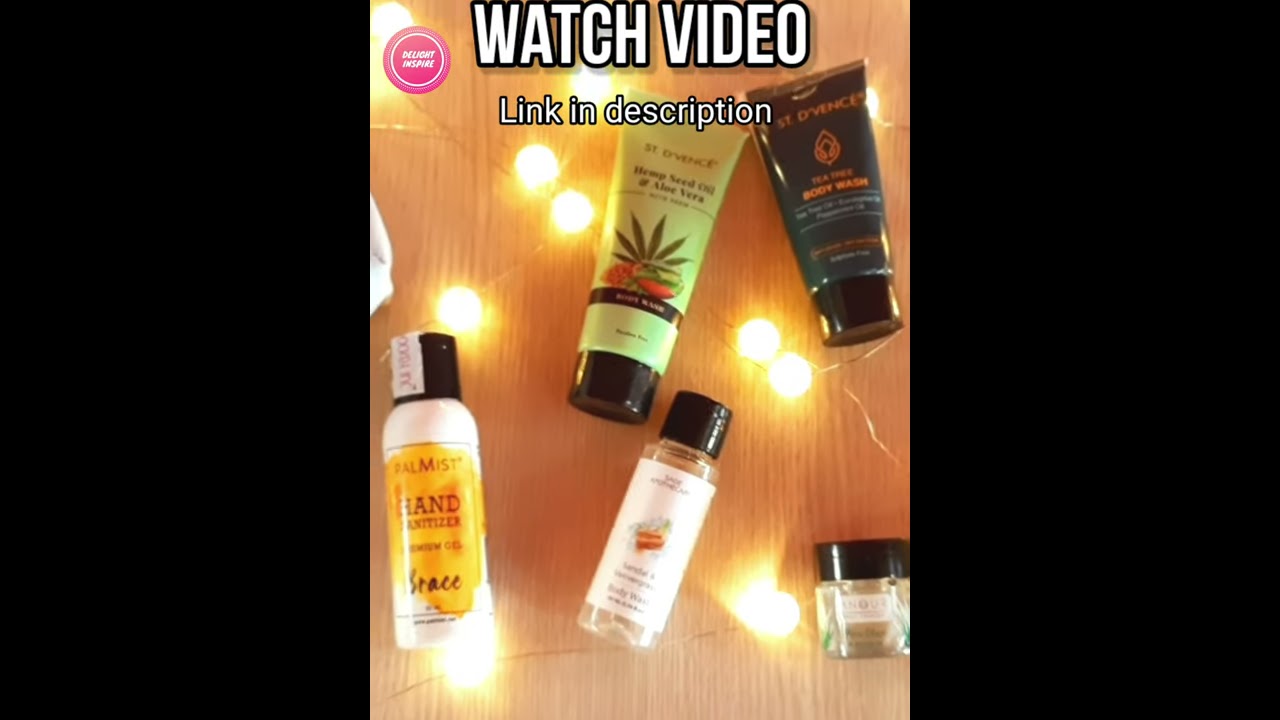The image showcases a centered photograph framed by black bands on the left and right sides. The photograph features a light brown wooden table that holds various toiletry products. At the top of the image, large white uppercase text outlined in black reads "WATCH VIDEO," with "link in description" in smaller white text below it. On the top left, there's a pink circle containing the text "Delight Inspire" in white, though it's slightly blurry.

The items on the table include a yellow squeeze tube with a black cap, adorned with a cannabis leaf graphic. To its right, a black squeeze tube with a black cap and gold lettering is visible. There are three bottles: a white plastic bottle with a black cap and a yellow label indicating "hand moisturizer" on the lower left, a smaller clear bottle with a black cap and a white banner beside it, and a green tube with leaf designs and a black cap above it. Another clear glass jar with a black screw top is positioned on the lower right. Also included are mentions of products such as hand seed oil with aloe vera, body wash, and hand sanitizer, though specific labels on some items are not entirely legible.